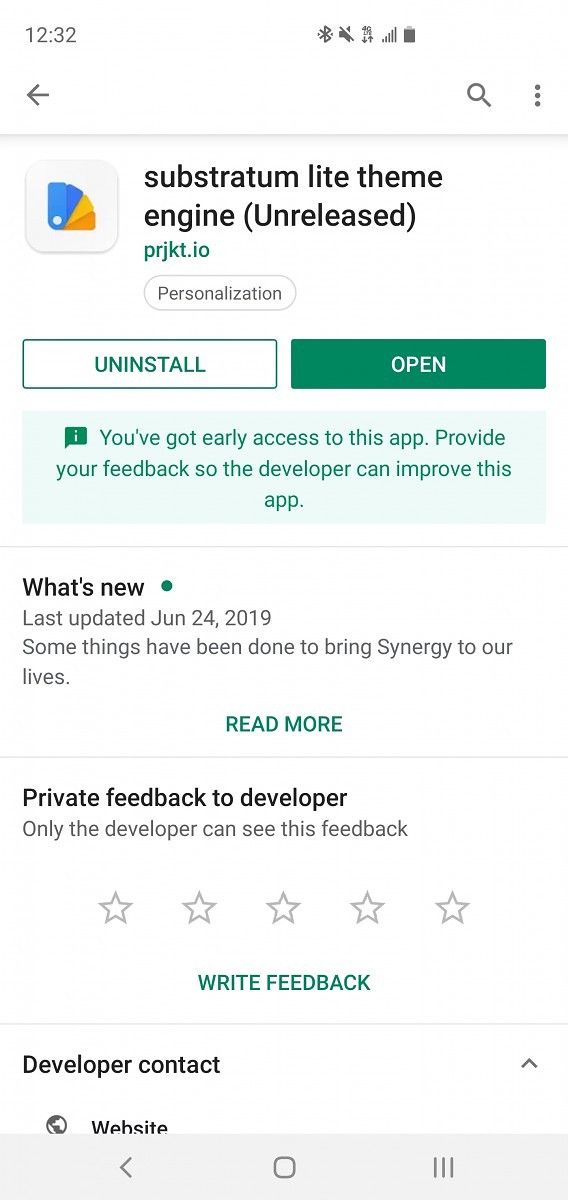This is a detailed screenshot of the Substratum Light Theme Engine app page on a cell phone. At the top, the text in black reads "Substratum Light Theme Engine (Unreleased)." A small blue hyperlink beneath it displays "prjkt.io," followed by the word "Personalization" in gray and small letters. Positioned underneath, there are two buttons: a white button with green text stating "Uninstall," and an identically sized button with inverted colors displaying "Open."

An accompanying icon, situated next to the title "Substratum Light Theme Engine," resembles a hand fan in yellow and blue hues. A notification in blue-green text informs the user that they have early access to this app with a request to provide feedback for improvement.

The next section, marked "What's New" in black text, reveals that the app was last updated on June 24, 2019, and mentions vague improvements aimed at bringing "synergy to our lives." A blue "Read More" link follows. Below, in black text, is a section for "Private Feedback to Developer," which notes that only the developer can see this feedback. This text is repeated once more.

Further down, there is an empty 5-star rating system, ready for user input, accompanied by a blue "Write Feedback" button. The final detail visible in the screenshot is a black "Developer Contact" text and a partial view of the word "Website" next to a small earth icon, indicating the presence of a web link for further information.